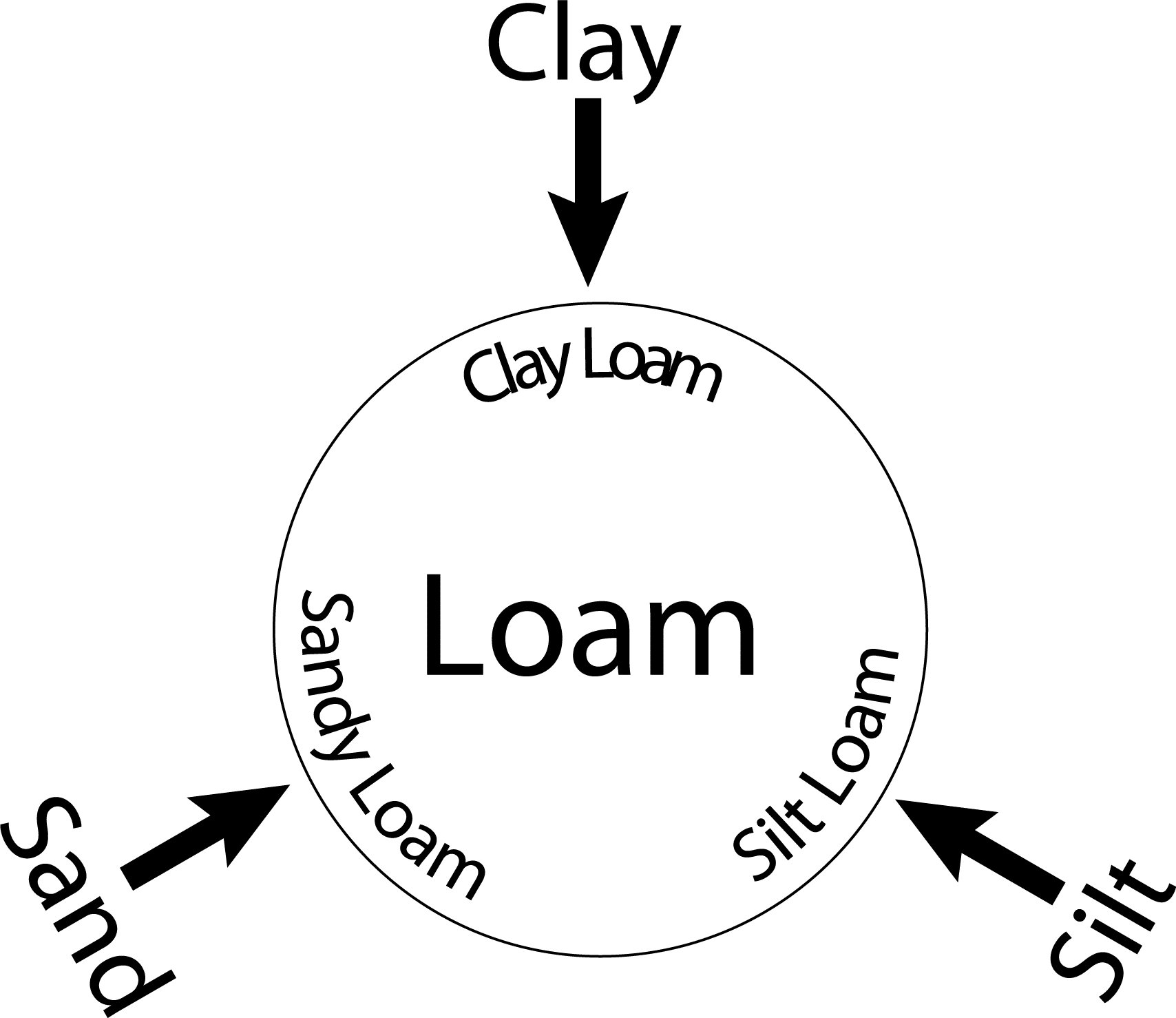This black and white infographic presents the composition and categories of loam soil. Central to the image is a large black circle labeled "loam" in prominent font. Within the circle, at the top (12 o'clock) position, is "clay loam," in the lower left (8 o'clock) position is "sandy loam," and at the lower right (4 o'clock) position is "silt loam." Outside the circle, three large words, "clay," "sand," and "silt," each paired with a black arrow, point towards their respective loam types. "Clay" is positioned at the top center, pointing to "clay loam;" "sand" is at the lower left, pointing to "sandy loam;" and "silt" is at the lower right, pointing to "silt loam." This detailed graphic effectively illustrates the different types of loam soil based on their primary components.